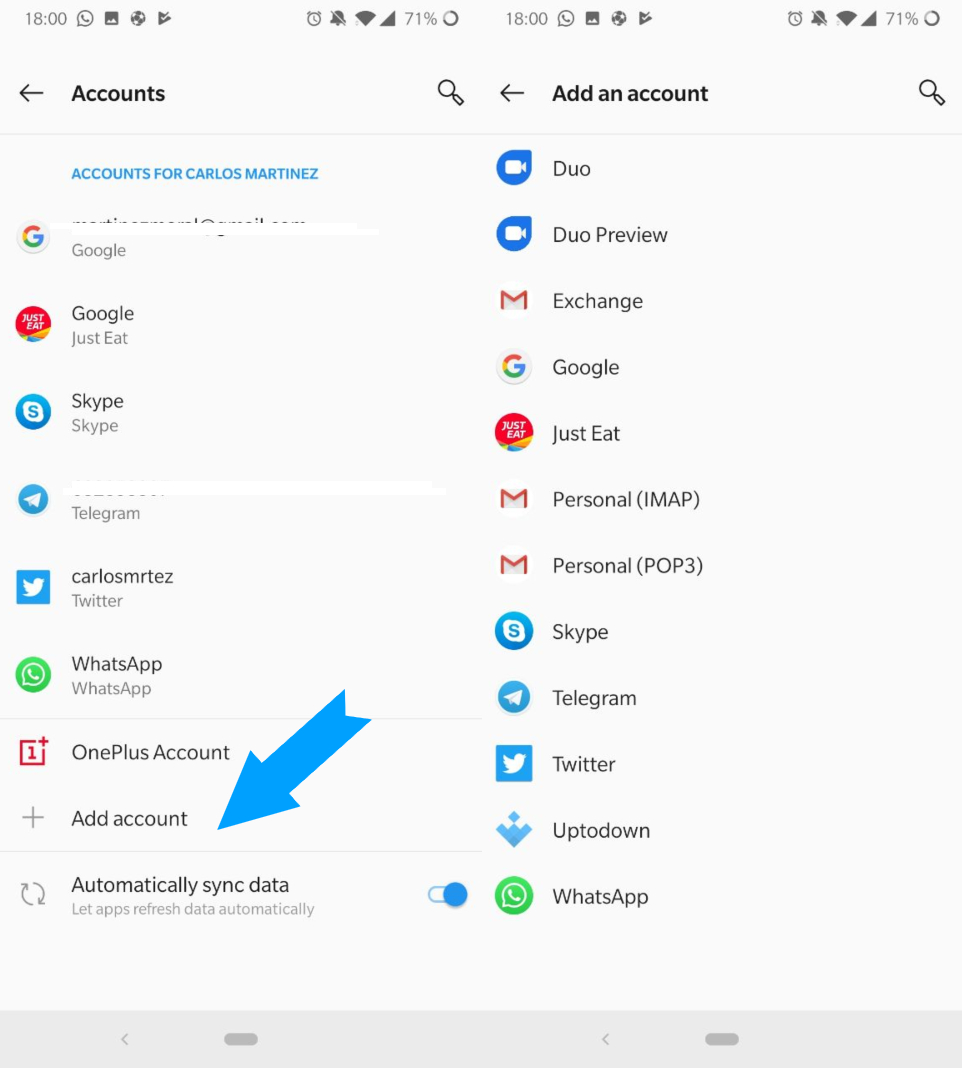This is a detailed description of a screenshot likely captured from a tablet, evident from its wide format or possibly two merged screenshots. The image showcases a settings menu for managing accounts. At the top, there are various app icons including WhatsApp, Gallery, Internet, and the Play Store.

On the left side of the screen, there is a section dedicated to accounts associated with Carlos Martinez. Below the header, "Accounts for Carlos Martinez," listed accounts include Google, Just Eat, Skype, Telegram, WhatsApp, and One Class Account. Additionally, there is an option to "Add Account," indicated by an arrow pointing to it, alongside an option to "Automatically Sync Data."

The right side of the screen features a separate list of account types, including Geo, Geo Preview, Exchange, Google, Just Eat, Personal Map, Personal POP3, Skype, Telegram, Twitter, UpToDown, and WhatsApp. The detailed account options and icons suggest a robust and organized user interface for managing multiple accounts on the device.